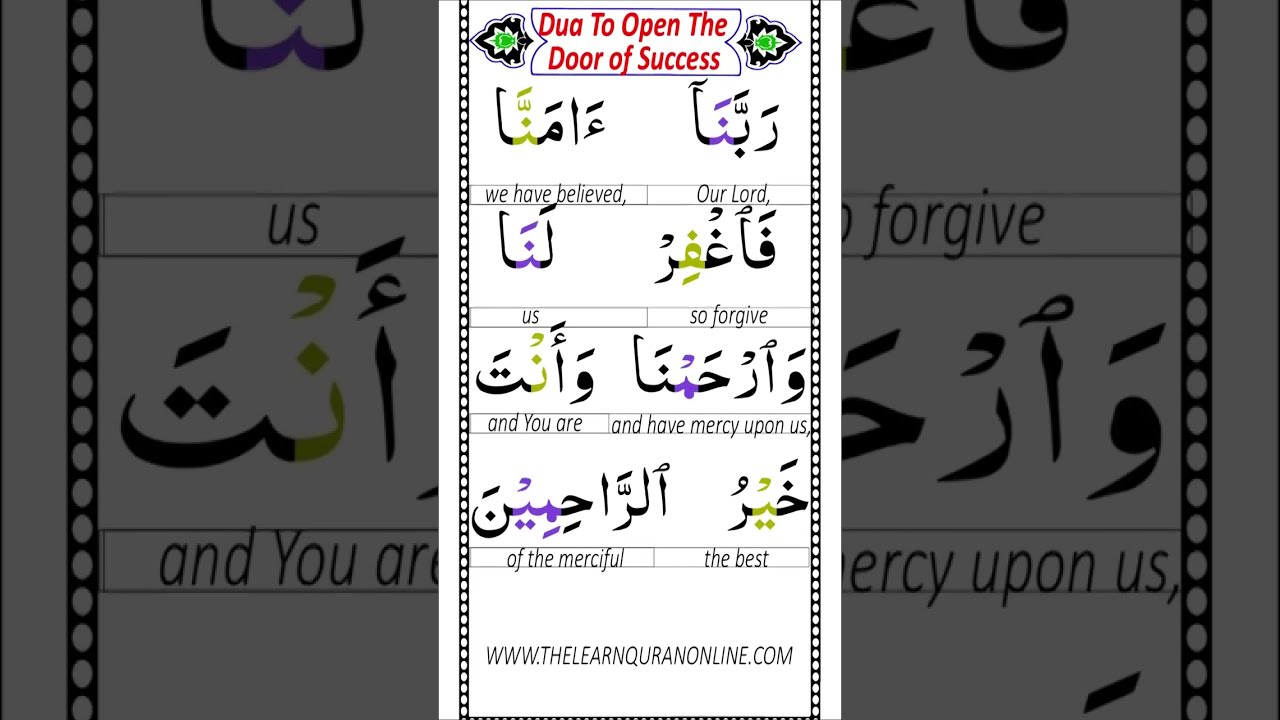The image is a vertical advertisement with a central, tall rectangular poster against a white background, framed by a black and white dotted border. At the top, in bold red italic letters, it reads "Dua to Open the Door of Success," flanked by decorative elements resembling arrowheads or curved leaves in black and green. Below the title, there is alternating Arabic script and English text. The Arabic script is depicted in black, purple, and light lime green colors. The English translations underneath read, "We have believed, Our Lord," followed by additional Arabic script, then "So forgive," more Arabic script, "And you are," further Arabic script, "And have mercy on us," and finally, more Arabic script that translates as, "Of the merciful, the best." At the very bottom, in black italicized text, the URL "www.thelearnquranonline.com" is displayed. The background subtly features a dark gray, zoomed-in, and stretched version of the central poster, creating a cohesive and engaging visual border.